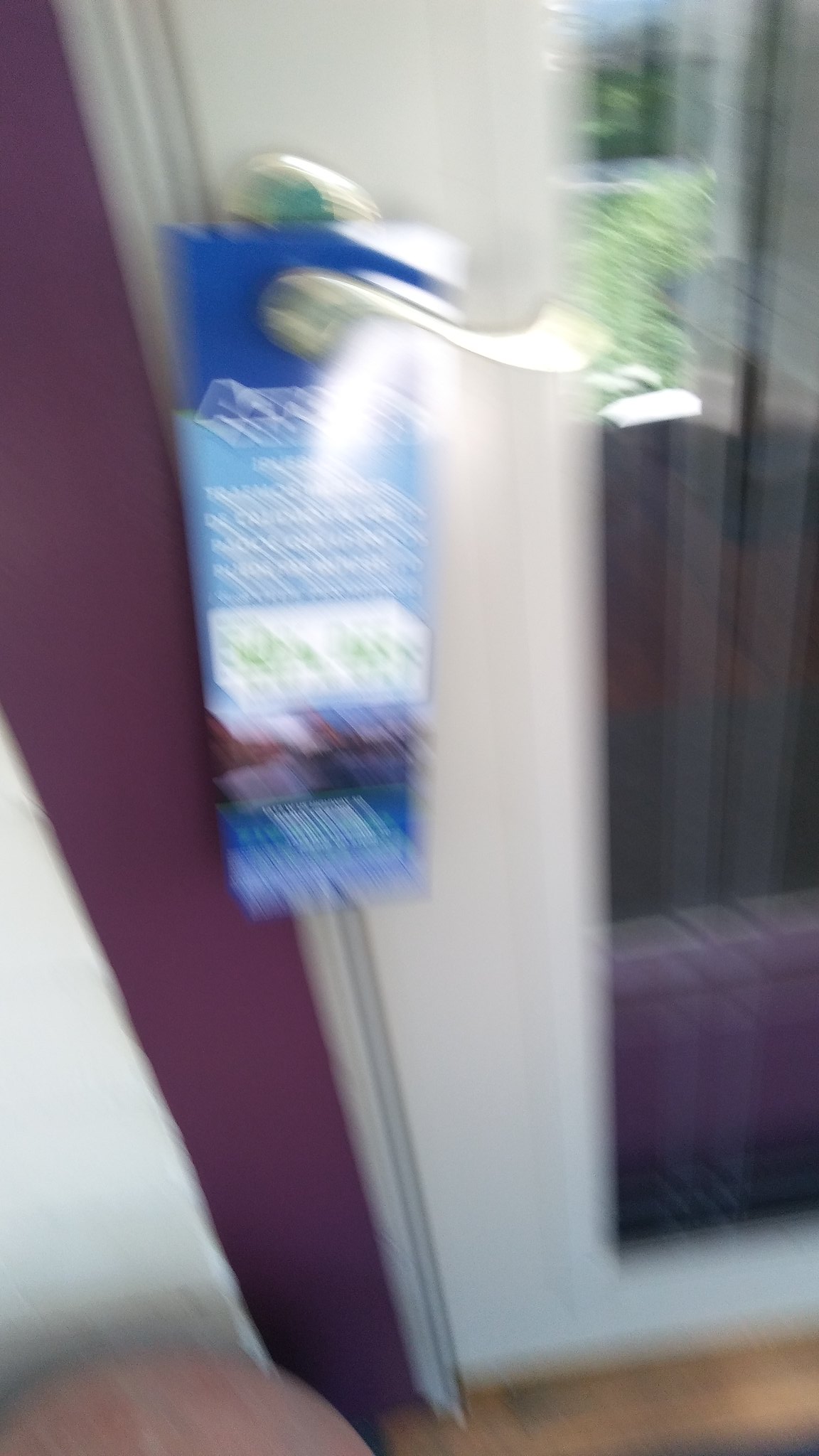This blurry vertical photograph depicts a white door situated in the center of the image, slightly ajar, with a gold door handle. Hanging from the handle is a distinctive label or card, featuring a dark blue top, light blue center, and a panel with white and green writing, likely similar to those "Do Not Disturb" signs seen in hotels. The surrounding walls are predominantly white, with a purple-hued wall section visible on the left. A reflective glass panel in the door reveals a glimpse of outdoor vegetation, suggesting a garden setting outside. The image also includes a brown floor at the bottom and a black window with hints of purple below it on the right, adding to the scene's overall complexity.